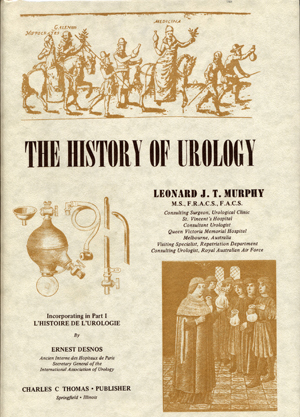The front cover of this book features a predominantly white and gray marbled background, presenting a classical, elegant aesthetic. The top section is adorned with a sepia-toned illustration capturing a medieval scene—a group of soldiers, some mounted on horseback and others walking. One figure rides side-saddle while others wear helmets and carry weapons, such as spears and swords sheathed at their sides. Shadows cast by their feet add depth to the image. Above this depiction are words that are unclear but integral to the composition.

Beneath this historical illustration, the title "The History of Urology" is boldly displayed in large, black letters. Midway down the cover, on the right side, the name Leonard J.T. Murphy, M.S., FRACS, FACS, a consulting surgeon in urology, is prominently listed, accompanied by additional professional details that highlight his credentials and background.

Adjacent to this text, a detailed diagram of a scientific apparatus is presented, consisting of a glass container with a spout, funnel, hose, and shutoff valve—evocative of plumbing or chemical equipment. The intricate diagram suggests a connection to the technical aspects of urology.

Below this apparatus, text describes "Incorporating in Part One, L. History de Urology by Ernest Desnos," indicative of a historical basis for the content. The publishing details follow, stating "Charles C. Thomas, Publisher, Springfield, Illinois."

Towards the bottom, another sepia-toned illustration mimicking the upper design features a man in a robe, possibly donning a wig, surrounded by several other men holding glass bottles, all dressed in medieval attire. This scene, placed above alternating-colored tiles, complements the overall historical theme of the cover.

This cover art, blending textual and illustrative elements, richly conveys the essence of a scholarly work on the history of urology.